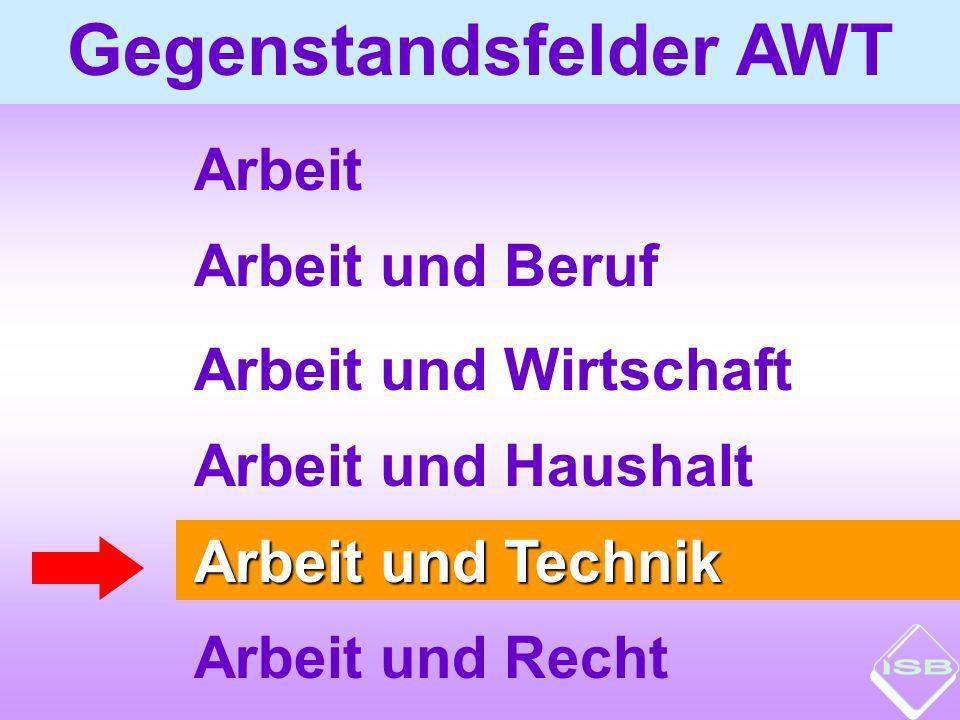The image is a detailed infographic poster predominantly in text, set against a background featuring a gradient of light lavender transitioning to white and back to a darker lavender. The upper part of the poster comprises a light blue horizontal bar with large, dark purple sans-serif text reading "Gegenstandsfelder AWT." Below this bar, the main body of the poster is centered horizontally and displays six lines of text, all left-justified in dark purple. The first line reads "ARBEIT," followed by "ARBEIT UND BERUF," then "ARBEIT UND WIRTSCHAFT," "ARBEIT UND HAUSHALT," and finally a line highlighted in an orange horizontal bar with shadowed text in white stating "ARBEIT UND TECHNIK," which has a red arrow pointing to it. The last line under this bar reads "ARBEIT UND RECHT." In the bottom right corner of the poster, there is a diagonally-tipped white diamond shape with the letters "ISB" inside. The language appears to be German, and the overall style is a blend of infographic design and typography.